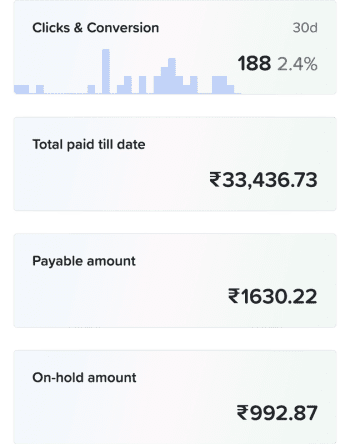The image displays a payment dashboard on a screen in a portrait orientation, divided into four equal sections. At the top section, titled "Clicks and Conversions," there's a 30-day overview represented by a bar graph. The graph features small ticks for each day, showcasing an up-and-down pattern with some days having no bars and others showing significant activity. The specific days are unlabeled on the axis.

Adjacent to the graph, the text indicates a total of 188 clicks and conversions, with a conversion rate of 2.4%. Below the graph, there's a summary stating, "Total Paid Till Date: 33,436.73," though the currency symbol is unclear—potentially British pounds.

Further details include:
- Payable Amount: 1,630.22 (same currency)
- On Hold Amount: 922.87 (same currency)

This comprehensive dashboard provides a financial snapshot, tracking clicks, conversions, and payment statuses over 30 days.